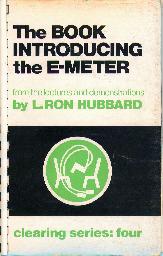This close-up image features the cover of an aged and weathered book with a paper binding, showing noticeable browning on the white edges. The title at the top of the book, printed in all caps in black text, reads: "THE BOOK INTRODUCING THE E-METER." Below the title, in green text, it states, "By L. Ron Hubbard." Centered on the cover is a black rectangle containing a green circle with a white outline. Inside the circle, there's an intricate design resembling two chairs connected by electrical wiring. At the bottom of the cover, more green text reads, "Clearing Series 4." The overall background of the book's cover is a clear white, contributing to its worn, antiquated appearance.